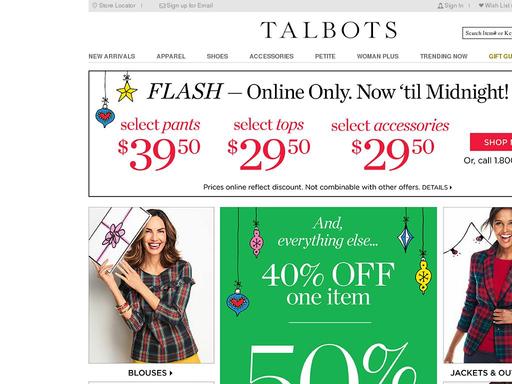The image features a promotional banner for Talbot's website with a gray header at the top displaying the text "Sign In." While part of the header text is blurry and unreadable, the clear elements include "New Arrivals," "Apparel," "Shoes," "Accessories," "Petite," "Woman," "Plus," "Trending Now," and "Gift."

Below the header, there are festive Christmas ornaments, including a star and a heart shape. Text beside these ornaments reads "Flash Online Only" and details the promotional period "Now till Midnight." Highlighted in red, promotional prices are listed as follows: "Select Pants - $39.50," "Select Tops - $39.50," and "Select Accessories - $29.50." A prominent red button below this information reads "Shop."

Further down, beneath the promotional offers, there is a note clarifying, "Prices Online Reflect Discount. Not combinable with other offers. Details."

A green box beneath the note contains two Christmas ornaments on the left and two on the right. It includes another promotional offer that states, "Everything Else - 40% Off One Item." Below this in text, "50%" is mentioned, though the context is not fully clear.

The overall image combines holiday-themed visuals with detailed promotional information aimed at encouraging online purchases.